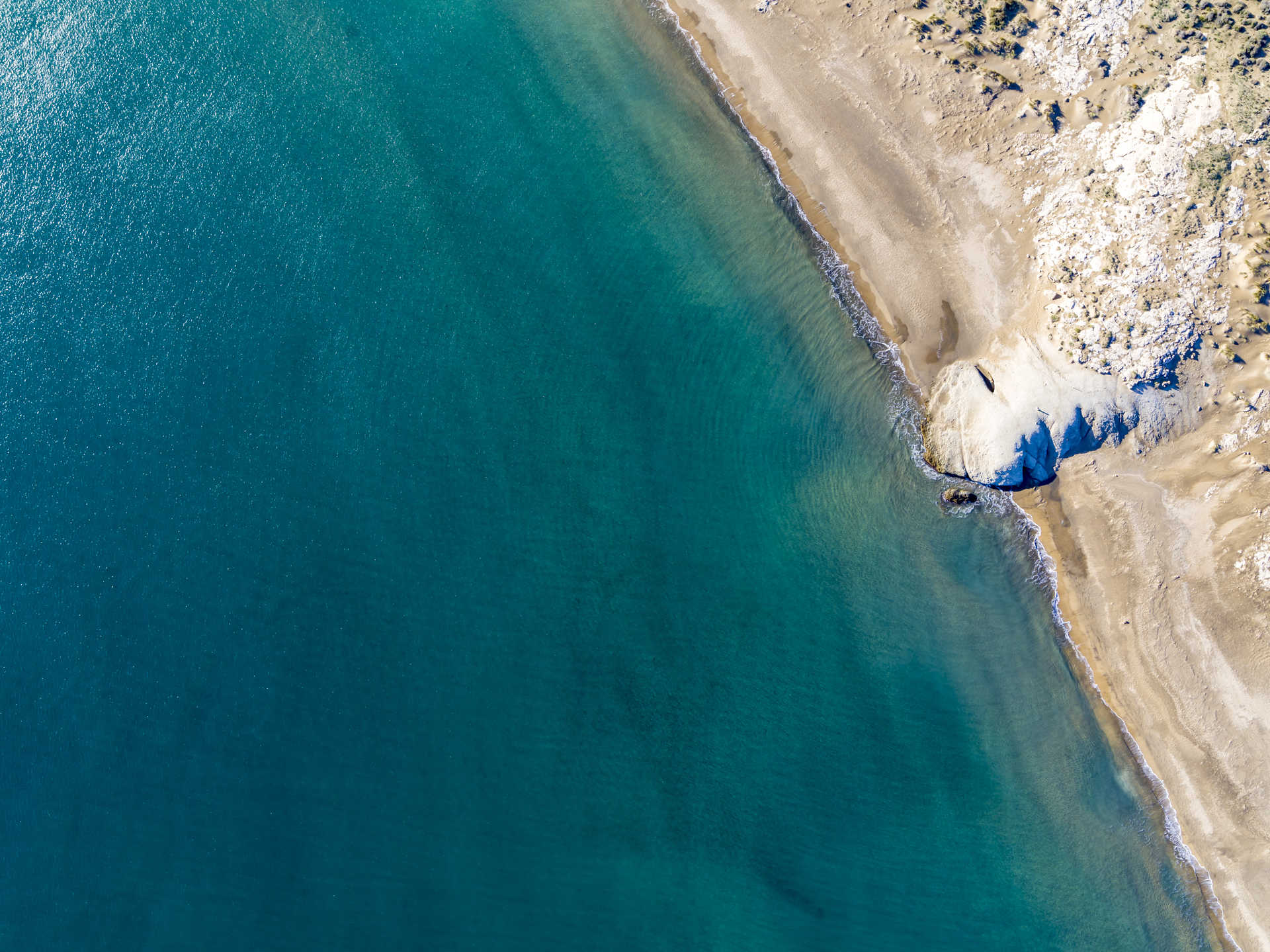An overhead shot captures a stunning beach scene dominated by a clear, teal-green ocean that spans more than three-quarters of the image. The sparkling water, dappled with sunlight, has a serene, calm appearance, with gentle ripples suggesting minimal wave activity, perhaps indicative of an island's tranquil shoreline. In the bottom right corner, a sandy beach emerges, with varying shades of brown indicating different levels of moisture. Along the shore, intricate rock formations and a substantial, white-topped rock structure jut from the landscape, creating a distinct J-shape. This prominent rock can be navigated around via shallow water or through a small, barely visible path connecting to the higher, hilly regions adorned with dried, white sand or salt.